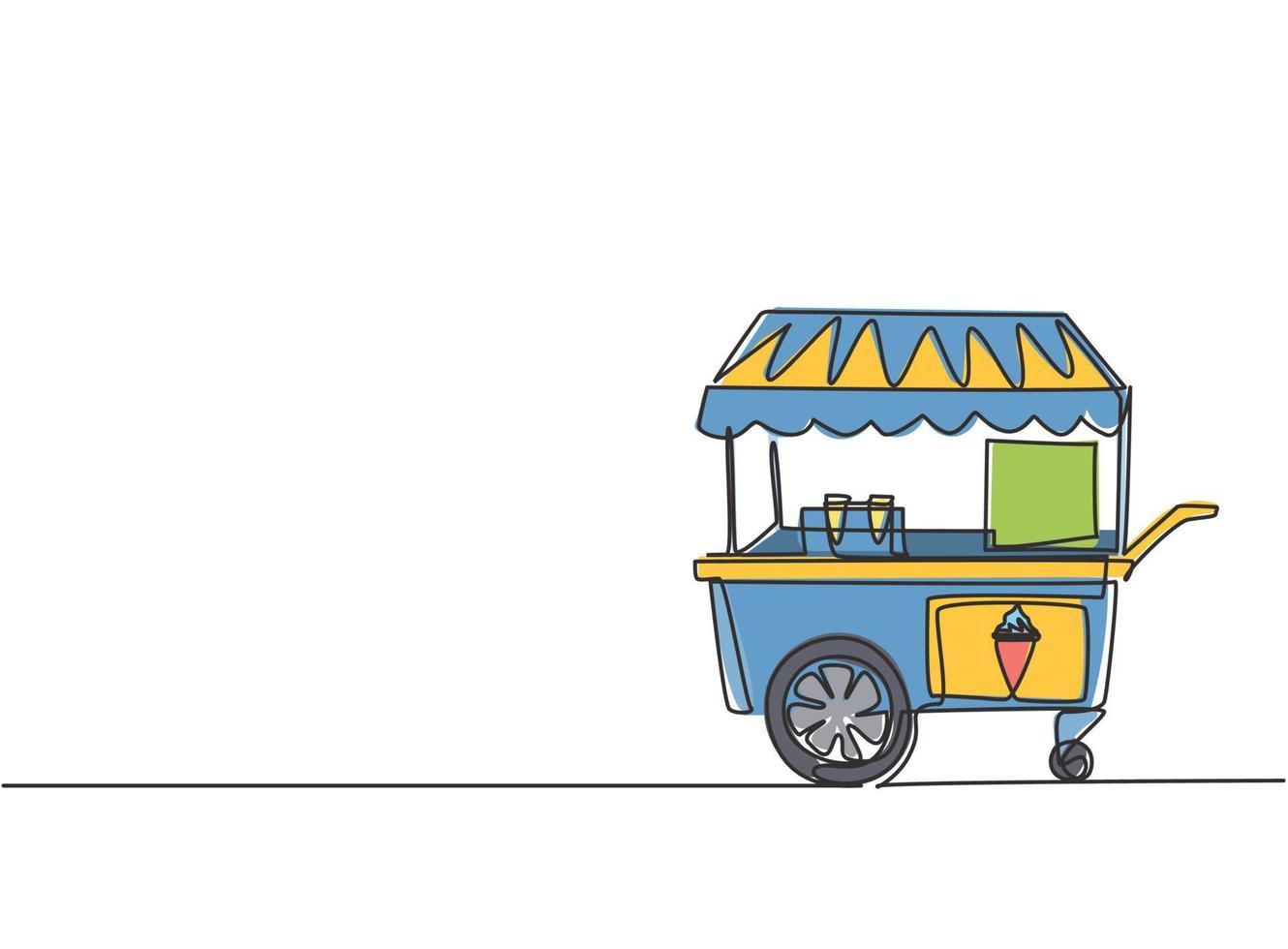This detailed image depicts a stylized, animated drawing of a mobile ice cream cart. The cart, primarily blue with yellow accents, stands out against a minimalist background. Across the bottom of the horizontal image runs a thin black line, simulating the surface on which the cart sits. The cart features two wheels: a small one at the front and a larger, black one with grayish spokes at the back. The cart's handle, which extends around the top, is a bright yellow, matching the triangular patterns on the blue awning above. 

On the cart's side, there's a colorful depiction of an ice cream cone with a pink cone and blue ice cream on top. Atop the cart, a green lid, presumably for accessing the ice cream, is lifted open, revealing cone holders and several ice cream cones inside. The scene is brightly lit with no visible human presence, focusing entirely on the vibrantly illustrated ice cream cart.